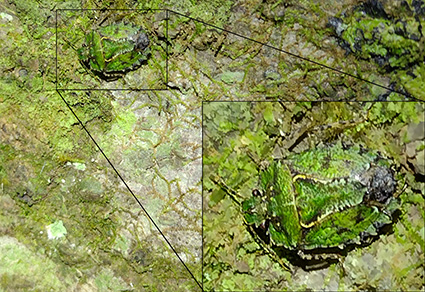This aerial photograph showcases a beetle skillfully camouflaged against a green and gray terrain. The beetle, positioned about a quarter of the way into the image from the top right, blends seamlessly with its surroundings due to its green and gray ridged shell. The shell, adorned with subtle white markings, is leaf-shaped—wide and tapering to a rounded point with small spikes along the edge.

To aid visibility, the photograph features a rectangular inset at the bottom right corner, providing a close-up view of the elusive insect. This inset is connected by lines from a black-outlined box drawn around the beetle in the main image. In the close-up, details such as two antennae and two eyes are distinguishable, emphasizing the beetle's intricate design and effective camouflage. The overall hue of the terrain and the beetle merge, enhancing the camouflage effect in this highly detailed imagery.